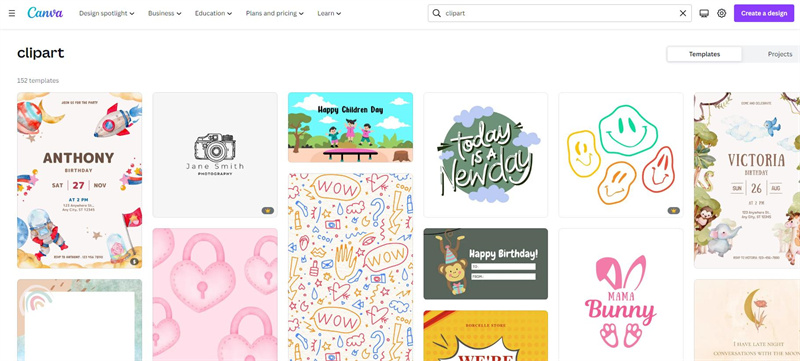This image showcases a Canva interface. At the top is the word “Canva” displayed in blue lettering. Below it, a search box shows a user has typed in "clipart", which has yielded 352 templates. 

Several templates are visible:

1. A template titled “Anthony” features black text with space-themed elements such as astronauts, flags, and spaceships.
2. Another template named “Jane Smith” displays a black drawing of a camera.
3. One captioned "Happy Children's Day" depicts children jumping on a bench at a park.
4. A piece of clipart with the text "Today is a new day" alongside uniquely shaped smiley faces, which are squiggly rather than round.
5. A template labeled “Victoria” with an adjacent partial image of a picture frame.
6. An image colored pink featuring pink locks.
7. A design with the word “Wow” adorned with handprints, hearts, and question marks.
8. A birthday-themed graphic with “Happy Birthday” and a monkey wearing a birthday hat.
9. A yellow template with a red stripe in the left corner, partially visible.
10. A graphic titled “Mama Bunny” in dark pink.
11. An image with balloon-themed clipart and unreadable text on a light pink background. 

This richly detailed interface highlights the diverse range of templates available for users to incorporate into their Canva projects.